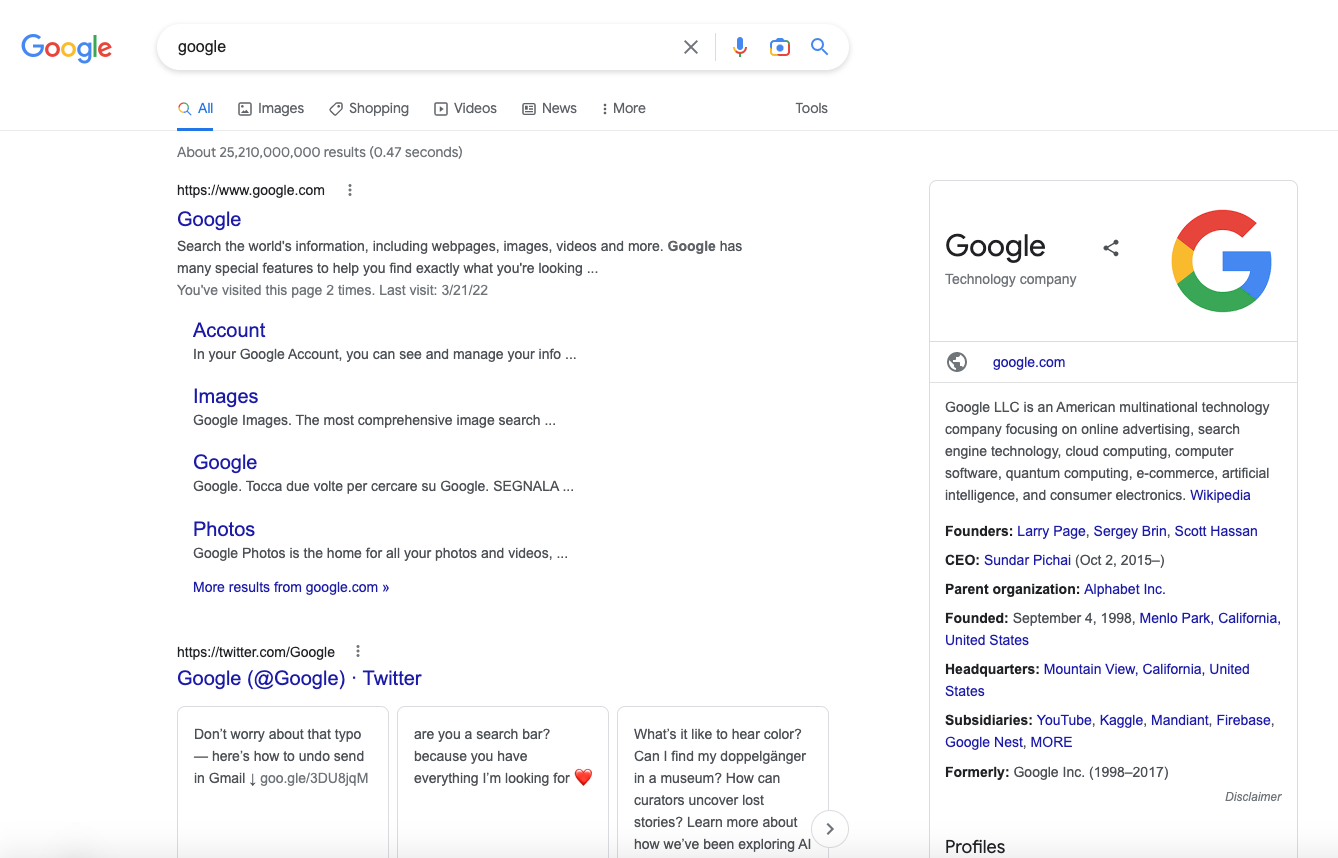This is a detailed caption for a photograph of a Google search results page:

The image displays a Google search results webpage, showcasing the iconic Google logo in its familiar blue, red, yellow, blue, green, and red colors prominently at the top. Beneath the logo, we see the search bar poised for a query, featuring a 'microphone' icon in blue, red, and green for voice searches, a 'camera' icon for visual searches, and a blue 'magnifying glass' to initiate the search. An 'X' icon is present to the right for clearing the search bar.

At the top of the page, the selected tab is "All," flanked by other search categories: "Images," "Shopping," "Videos," "News," and "More." To the right of these options is the 'Tools' bar, offering additional filtering options. The results section indicates an impressive total of 25,210,000,000 results, rendered in just 0.47 seconds, reflecting Google's efficiency.

Near the top, "Google" is written in bold blue font, aligning with other text elements such as 'Account,' 'Images,' 'Google,' and 'Photos,' which are repeated for navigational purposes. A Twitter handle labeled 'Google' is spotted, suggesting social media integration.

The right side of the page provides quick biographical snippets about Google's founders—Larry Page, Sergey Brin, and Scott Hassan—highlighting Google's roots as a pioneering technology company. The clean, colorful interface utilizes Google's traditional color scheme, enhancing both functionality and visual appeal.